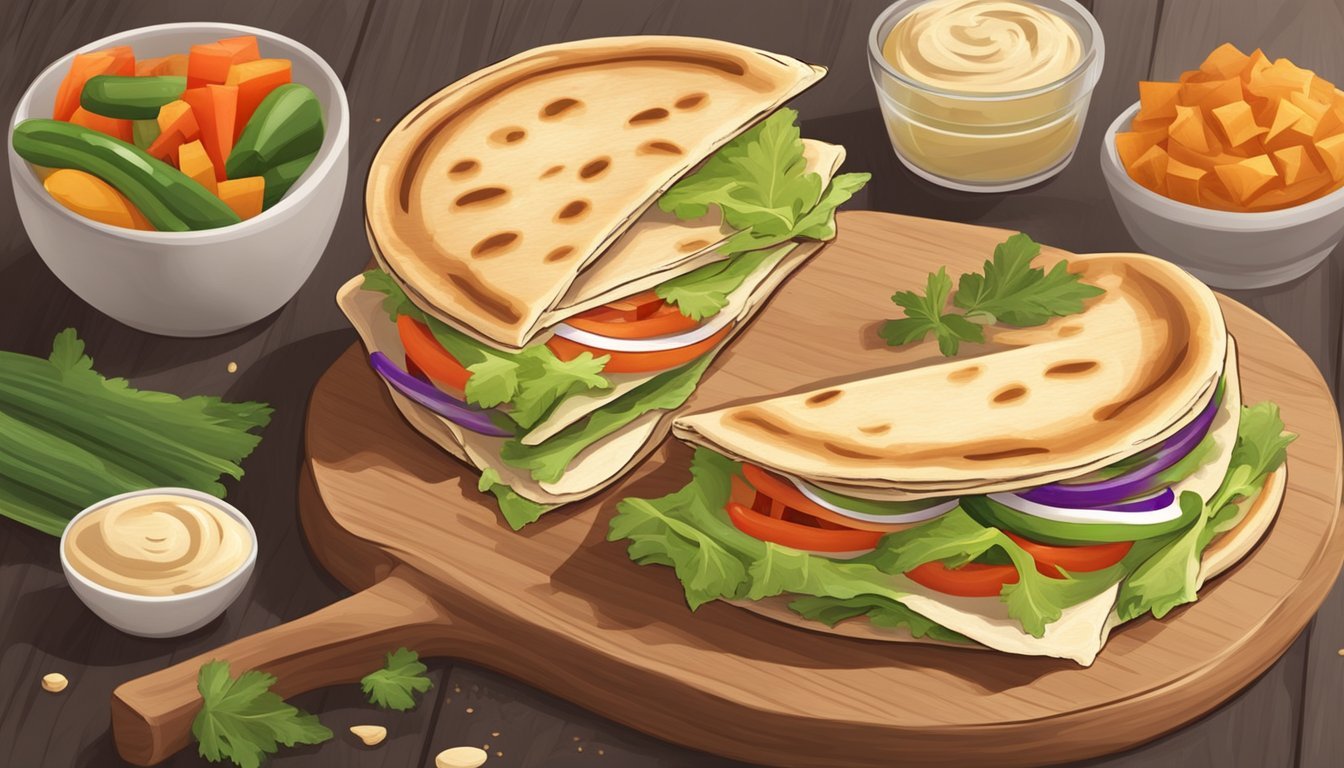This is a digital illustration of a food scene featuring a pita sandwich cut in half on a light brown wooden cutting board. The sandwich, which appears toasted, is layered with lettuce, tomatoes, red onions, and possibly cheese. Surrounding the board are various dishes and ingredients: 

- To the upper left, there is a white ceramic bowl filled with mixed vegetables including carrots and cucumbers.
- Below that bowl, there are sprigs of fresh green herbs, likely cilantro or parsley, and a small white bowl containing a creamy white sauce, possibly hummus.
- On the top right, a larger glass bowl containing beige hummus sits next to a white ceramic bowl filled with chopped sweet potatoes or carrots.
- On the left side, another small bowl of hummus is present alongside some celery stalks.
- Scattered pieces of parsley or cilantro are also visible, with a noticeable spill of the white sauce at the bottom left of the image.

The entire scene is set on a dark wooden table, adding a rustic feel to the vibrant and detailed composition.